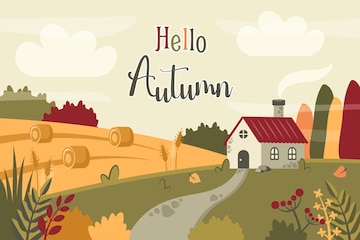This digital graphic illustrates a charming, almost cartoonish autumn scene centered around a single cottage perched on a hillside. The cottage, resembling a one-room schoolhouse, features a distinct red tile roof and a chimney. A winding path leads up to it from the bottom of the image. The entire environment is adorned with rich fall hues of red, orange, and soft yellow. To the left of the house lies a green, rolling field filled with round haystacks, indicative of a recent harvest. Surrounding the scene are various trees, their foliage displaying a vibrant mix of green, yellow, red, and peach. In the sky, there are clouds that give an impression of a gentle breeze blowing through. The center of the graphic prominently features the text "Hello Autumn," encapsulating the seasonal theme. Both the right and left corners of the image are dotted with plants, completing the idyllic fall landscape.